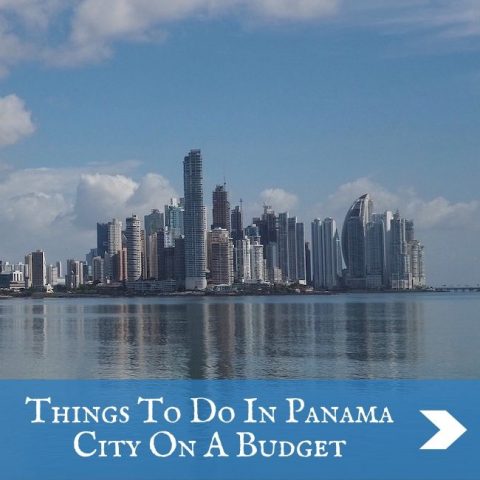The image captures a vibrant cityscape under a bright blue sky dotted with puffy white clouds. In the center of the photograph, a bustling city skyline rises from a strip of land, featuring tall buildings of varying heights reflecting in the light blue water below. The shoreline serves as a boundary between the urban structures and the tranquil expanse of water, which beautifully mirrors the cityscape. 

Just below this picturesque scene, there is a thick blue rectangle occupying less than a quarter of the image. Inside the rectangle is a crisp white text that reads: “Things to do in Panama, City on a Budget.” To the right of this text, there is a bold white chevron arrow pointing to the right, directing attention forward.

Further enhancing the photograph's detailing, a dark patch is visible in the water, resembling a dark rectangle. This patch is caused by the reflection of some of the darker concrete buildings, adding depth and contrast to the overall serene and reflective water surface.